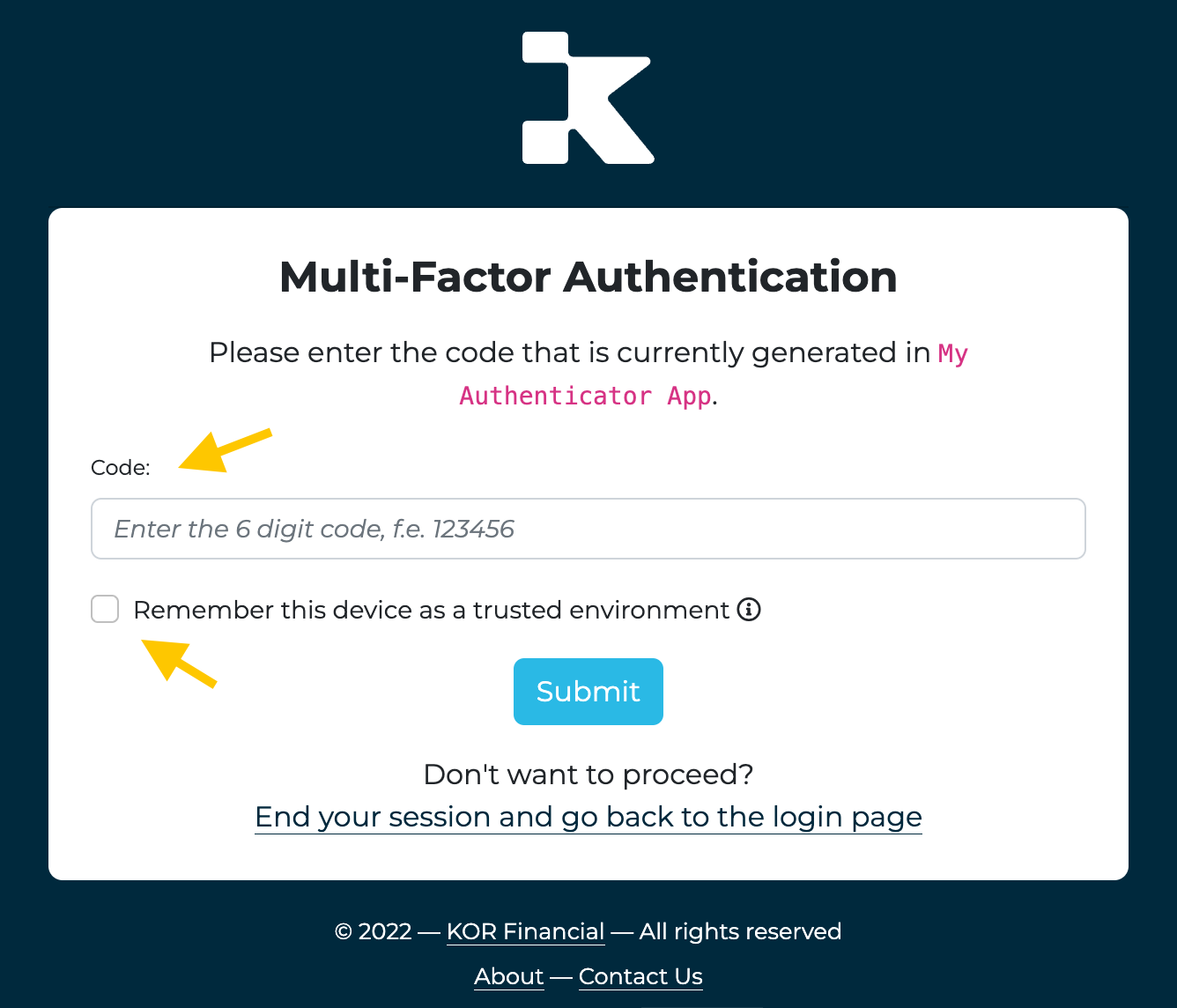The image displays a screenshot of a digital authentication page, likely viewed on a computer or a phone. At the top, there is a stylized "K" logo with a small chunk missing from the upper part. Below the logo, within a centrally placed white rectangle set against a black, square-shaped background, the text "Multi-Factor Authentication" is prominently displayed in black print.

The main section of the page prompts the user with the message: "Please enter the code that is currently generated in My Authenticator app." Beneath this instruction, a labeled input field reads "Code," adjacent to a blank space meant for the six-digit code entry. The text "Enter the six-digit code, e.g., 123456" is provided as an example.

A yellow arrow points down towards the "Code" input area, drawing attention to it. Further down, there is a checkbox with the label "Remember this device as a trusted environment," accompanied by an encircled lowercase "i" providing additional information.

At the bottom, a second yellow arrow directs attention to a blue button labeled "Submit" in white print. Additional text underneath the button offers an option for users who do not wish to proceed: "Don't want to proceed? End your session and go back to the login page."

The footer of the page includes a copyright notice, "© 2022," followed by links labeled "About" and "Contact Us."